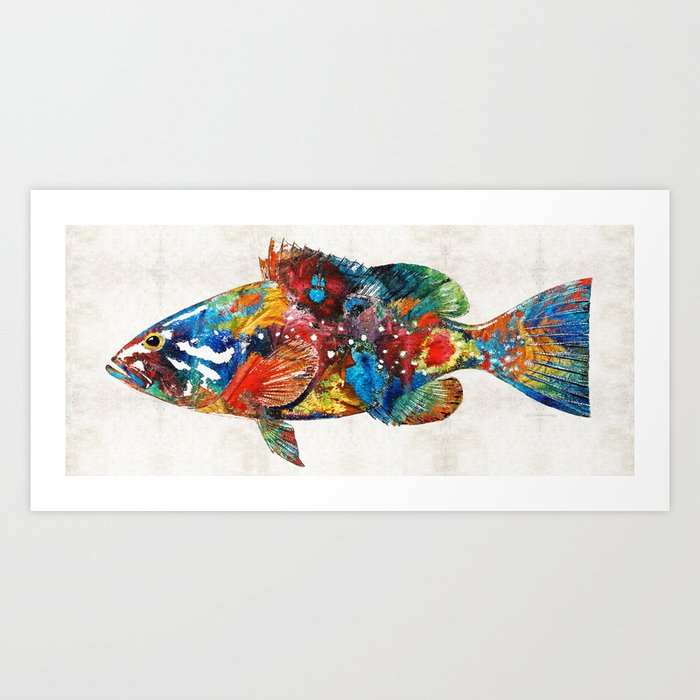The image showcases a vibrant and detailed piece of artwork depicting a side profile of a fanciful fish. Mounted on a light gray wall, the artwork features a white trim surrounding a patterned grayish background that highlights the colorful fish. The fish itself is an explosion of colors, including shades of red, blue, green, yellow, orange, turquoise, and white, creating a unique and non-naturalistic pattern. The fish has a large black eye circled with yellow and a prominent mouth, suggesting it might be an ocean-going species. Its small dorsal fin transitions from orange to red to blue, while a rounded fin behind it fades from dark blue to medium green. The head of the fish starts with a red hue, followed by a blue stripe on the bottom jaw. The colors transition into blues and greens across the body and include yellows, oranges, and burgundy, creating a dynamic and visually captivating design. The wide tail primarily features blues, accented with oranges, yellows, red, and white. This striking illustration, potentially done in watercolor, is designed to stand out with its rich and varied palette that extends across the entire fish.